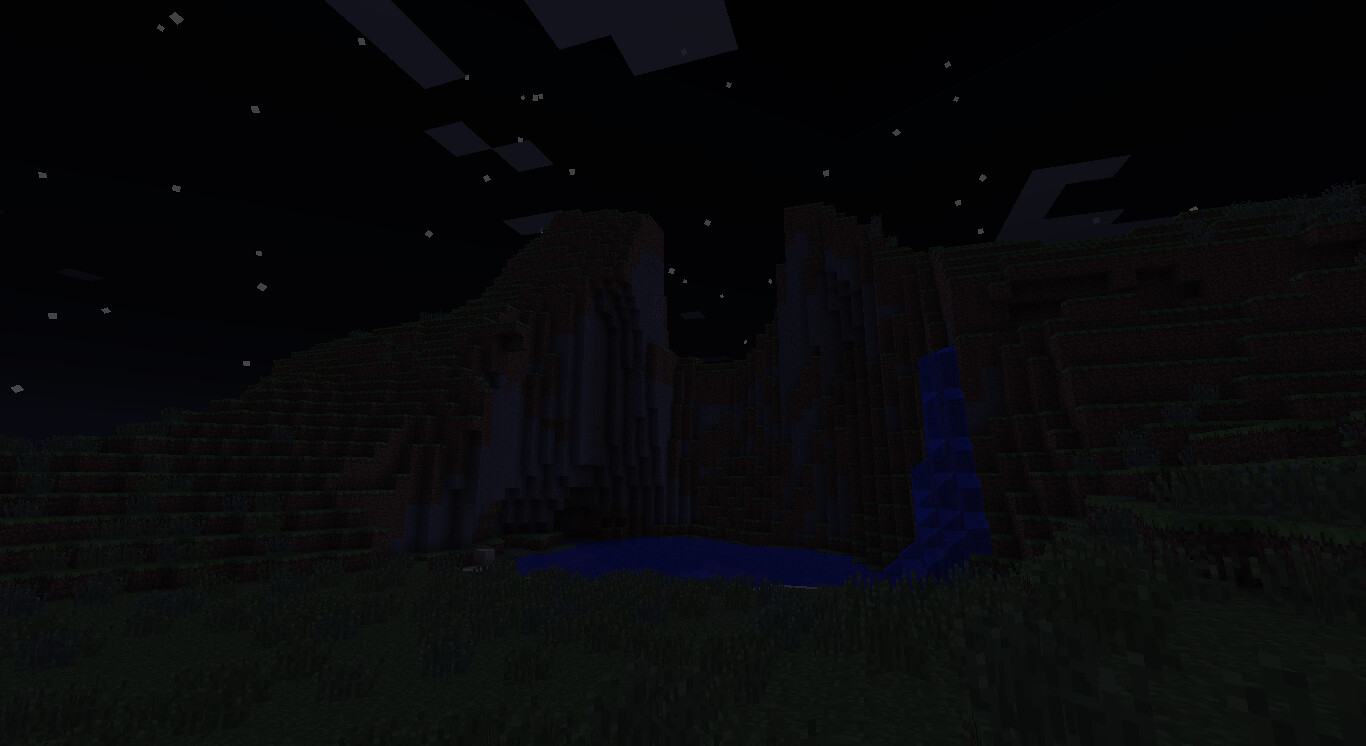"A mysterious rectangular black square dominates the frame, void of any discernible image. Despite multiple attempts to upload the original content, it seems this black square is all that remains. Upon closer inspection, there might be a subtle hint of blue peeking through the inky darkness, though it could be a trick of the eye or even a speck of dirt on the screen. The longer you gaze into the abyss, the more your eyes try to find meaning in the emptiness."